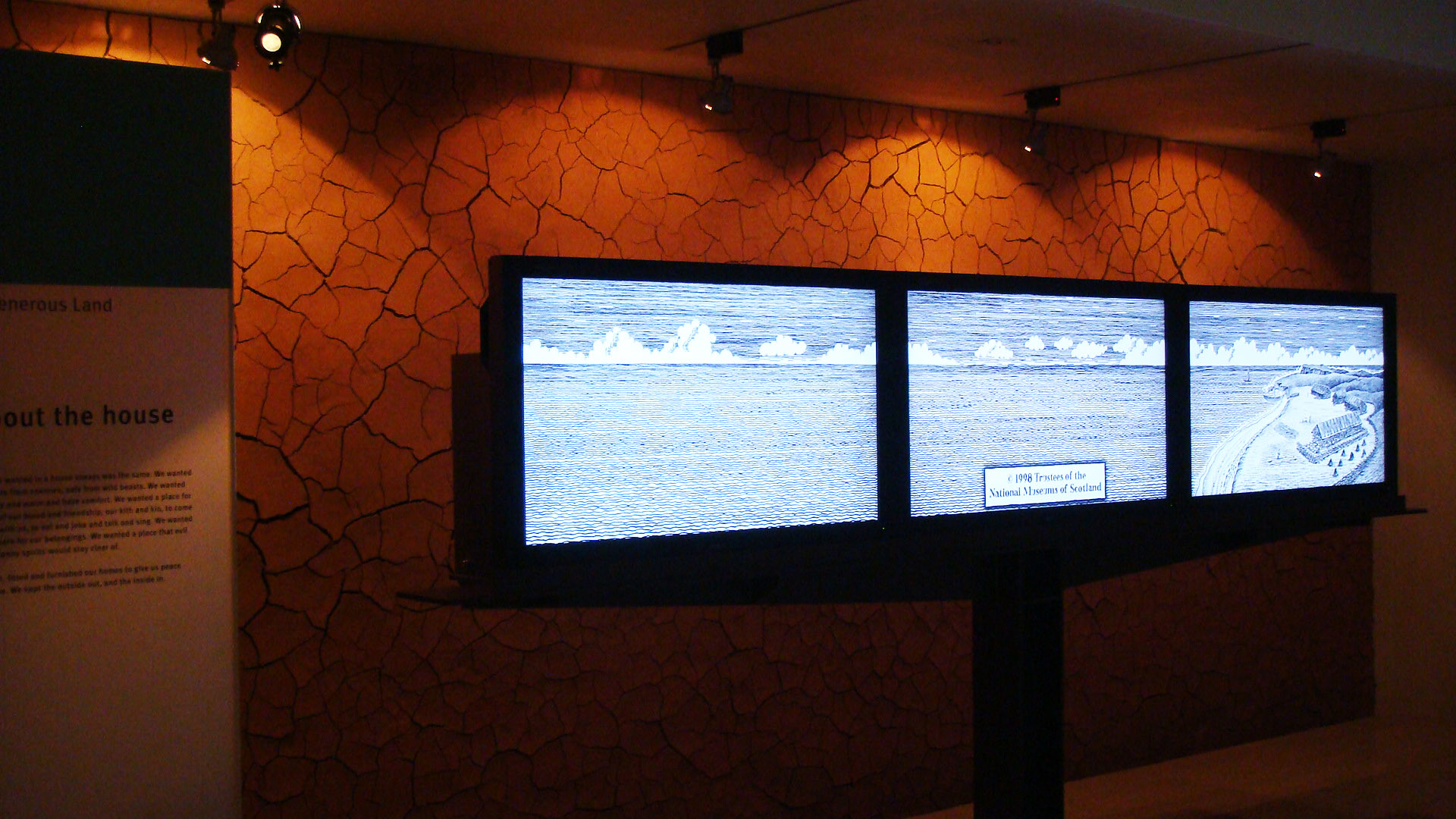The image displays a dimly lit indoor museum exhibit highlighting a coastal scene across three large TV screens mounted on a black pedestal platform. The screens collectively depict a seamless panorama of a blue ocean with waves, extending from the left to the right. On the rightmost screen, the scene transitions to a grassy area with a wooden hut and trees, suggesting a coastal village. Above the screens, there are four spotlights casting light down onto a textured, cracked, orangey-brown wall that resembles dried desert earth. In the middle screen, text reads "1998 Trustees of the National Museums of Scotland." To the left, there's a partially visible banner with the words "Out the House," and a text panel providing exhibit information. This exhibit captures the essence of a tranquil shoreline bordered by an antiquated village.